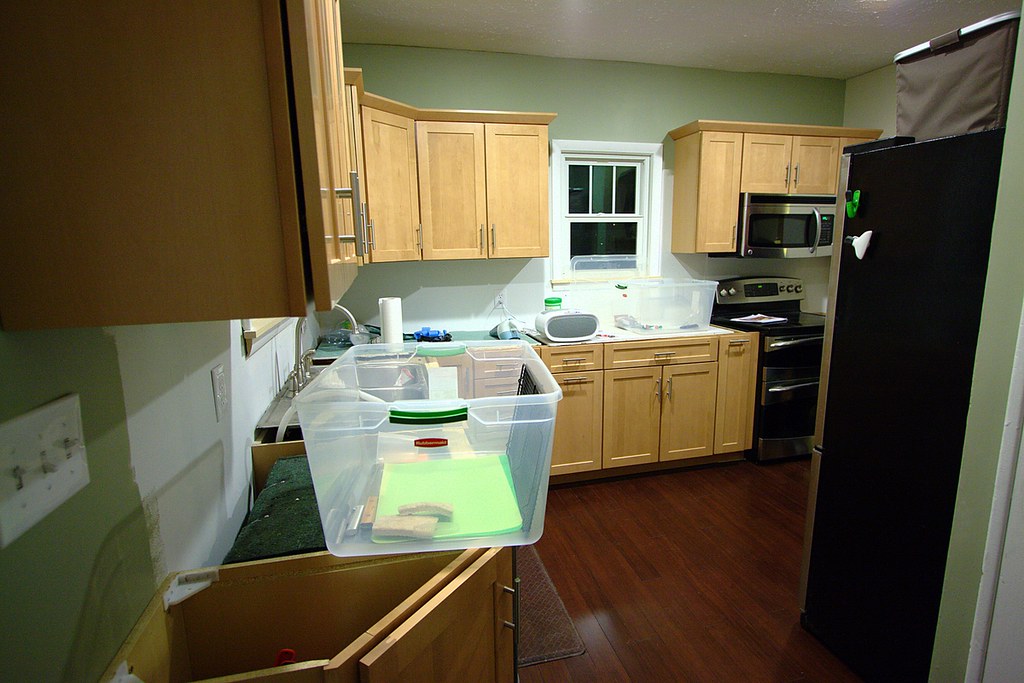This detailed photograph captures a traditional American kitchen under renovation. The walls are painted a muted olive green, providing a warm and earthy backdrop. The cabinetry is made of rich pine wood, adding a touch of natural elegance. The floor is composed of cherry or walnut-stained wood, complementing the cabinets with its darker, polished hue. On the right side of the image, a sleek refrigerator is visible, featuring black sides and a stainless steel front. Adjacent to the refrigerator is a modern range with black and stainless steel finishes, over which a matching microwave is built into the surrounding cabinetry. To the left of the range, there's a window above the sink that lets in natural light. The countertops are cluttered with various items, including several Rubbermaid containers, a roll of paper towels, and some napkins, partially obscuring the surface beneath. Notably, part of the counter appears to be missing, indicating ongoing construction or renovation. The image is crisp and clear, devoid of any people or text, focusing solely on the kitchen and its current state.